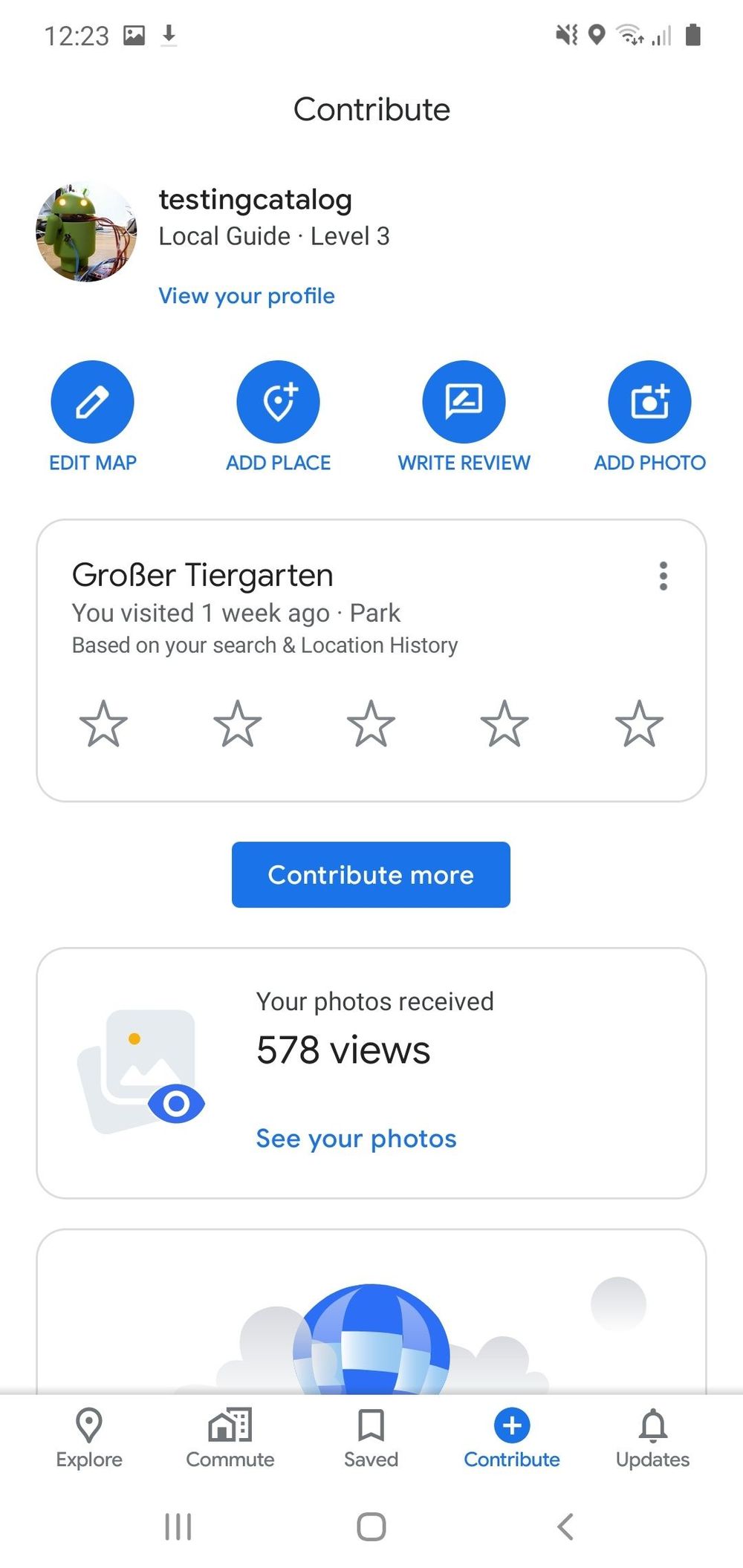This image depicts a smartphone interface, specifically a contribution page for a local guide application. The top right corner shows standard phone icons such as battery life and connectivity status, with the current time reading 12:23. Dominating the top section is the word "CONTRIBUTE" in bold black letters. Directly beneath it, the screen indicates "Testing Catalog" followed by "Local Guide: Level 3". Adjacent to this text is a small, digitized green character. Below, a clickable blue link reads "View Your Profile".

The main section features a grid of four large icons: "Edit Map," "Add Place," "Write Review," and "Add Photo," presumably options for user contributions. A white box with gray borders displays "Grover Tiergarten," noting this location was visited one week ago. It mentions that it is a park based on search and location history. This section also shows five empty stars, indicating that the location has not yet been reviewed. At the top right corner of this box are three vertical dots for additional options.

Further down, a blue button with the text "Contribute More" encourages additional user interaction. Another gray-bordered box states "Your photos received 578 views," with a clickable link "See Your Photos" in blue text. An adjacent icon of an eye suggests the visibility of the photos.

The interface's bottom navigation bar includes options labeled "Explore," "Commute," "Saved," "Contribute," and "Updates", providing easy access to different sections of the app.